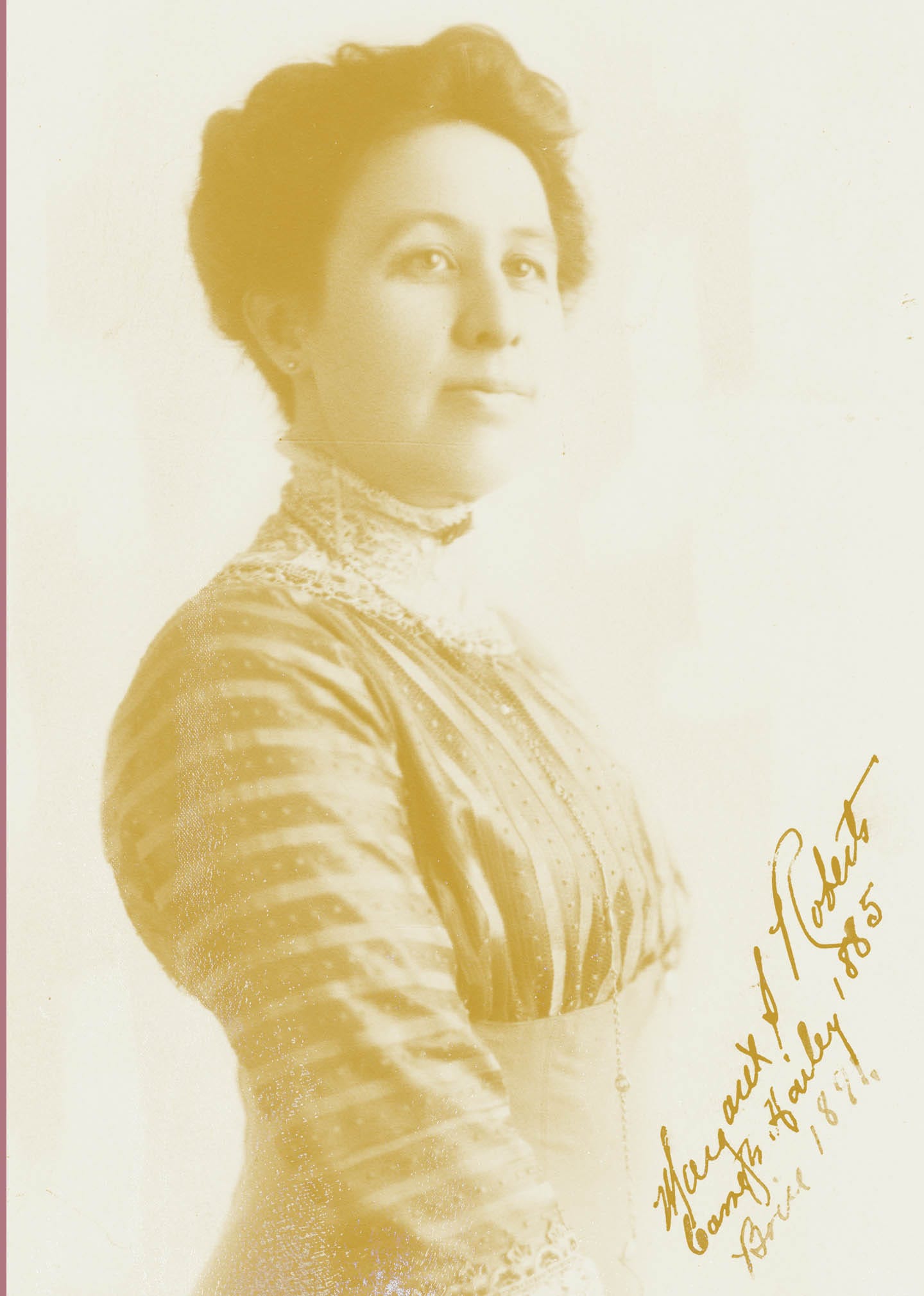This portrait photo, approximately one and a half times taller than it is wide, is a washed-out black and white image dated either 1885 or 1894, according to the cursive signature in the lower right corner which remains partially illegible. The photo captures a woman with short, curly brown hair styled up, adorned with earrings visible in her right ear. She faces slightly to the right of the camera, with her gaze directed slightly down and away. Her expression is bright, showcasing her fuller cheeks and lively eyes.

The woman is dressed in period clothing typical of the late 19th century. She wears a striped shirt with darker stripes between lighter ones, detailed with lace that extends up her neck and decorates her sleeves. The shirt appears to have polka dot patterns interwoven with the stripes, adding to the ornate design. A white lace collar, resembling doilies, complements her bustier or corset at the bottom. Her complexion is light, possibly indicative of being a white woman or having a light brown complexion, as some interpretations vary. The image captures her from the waist up, providing a detailed view of her intricate attire and her elegant demeanor.